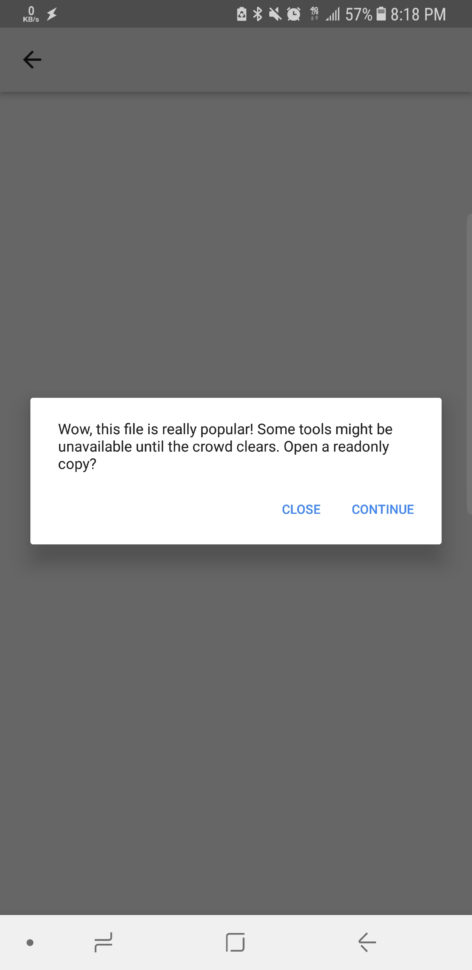In the screenshot of a cell phone display, we observe a crucial pop-up window prominently centered on the screen. The pop-up is enclosed in a white box with black text, delivering an important message that states: "Wow, this file is really popular. Some tools might be unavailable until the crowd clears. Open a read-only copy." Notably, the phrase "read-only" is written as a single concatenated word. Below this message, in the bottom right corner of the pop-up, there are two actionable buttons labeled "Close" and "Continue."

The backdrop of this white pop-up window is a gray screen. This gray background hosts cell phone icons arrayed in a darker gray bar at the top of the screen, stretching horizontally from left to right. Beneath this darker gray notification bar lies another bar, this time occupied by a 'back' arrow on the left-hand side.

The timestamp displayed on the phone reads 8:18 PM, which is visible at the bottom right corner of the screenshot, further enhancing the contextual details of the image.